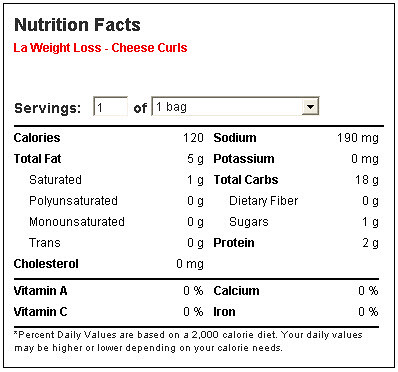This computer-generated image displays the nutrition facts for "LA Weight Loss Cheese Curls" in a consistent, box-like format. Positioned prominently in the top left corner, the title "Nutrition Facts" is printed in bold black text. Beneath it, the product name "LA Weight Loss Cheese Curls" is indicated, suggesting that this label provides detailed nutritional information for a serving of cheese curls specifically catered to weight loss programs.

The label is comprehensive, outlining various nutritional components: it specifies the serving size and the total calorie count per serving. It breaks down the total fat content, including subcategories for different types of fats, such as saturated and trans fats. Additionally, the label lists cholesterol, sodium, potassium, and total carbohydrate content, the latter further detailed into dietary fiber, sugars, and proteins.

At the bottom of the label, it also notes the presence (or absence) of essential vitamins and minerals, indicating that the product has 0% of the daily recommended value for Vitamin A, Vitamin C, calcium, and iron. Finally, the label includes explanatory information regarding percent daily values, providing context for how these values contribute to an individual's daily nutritional requirements based on a standard diet.